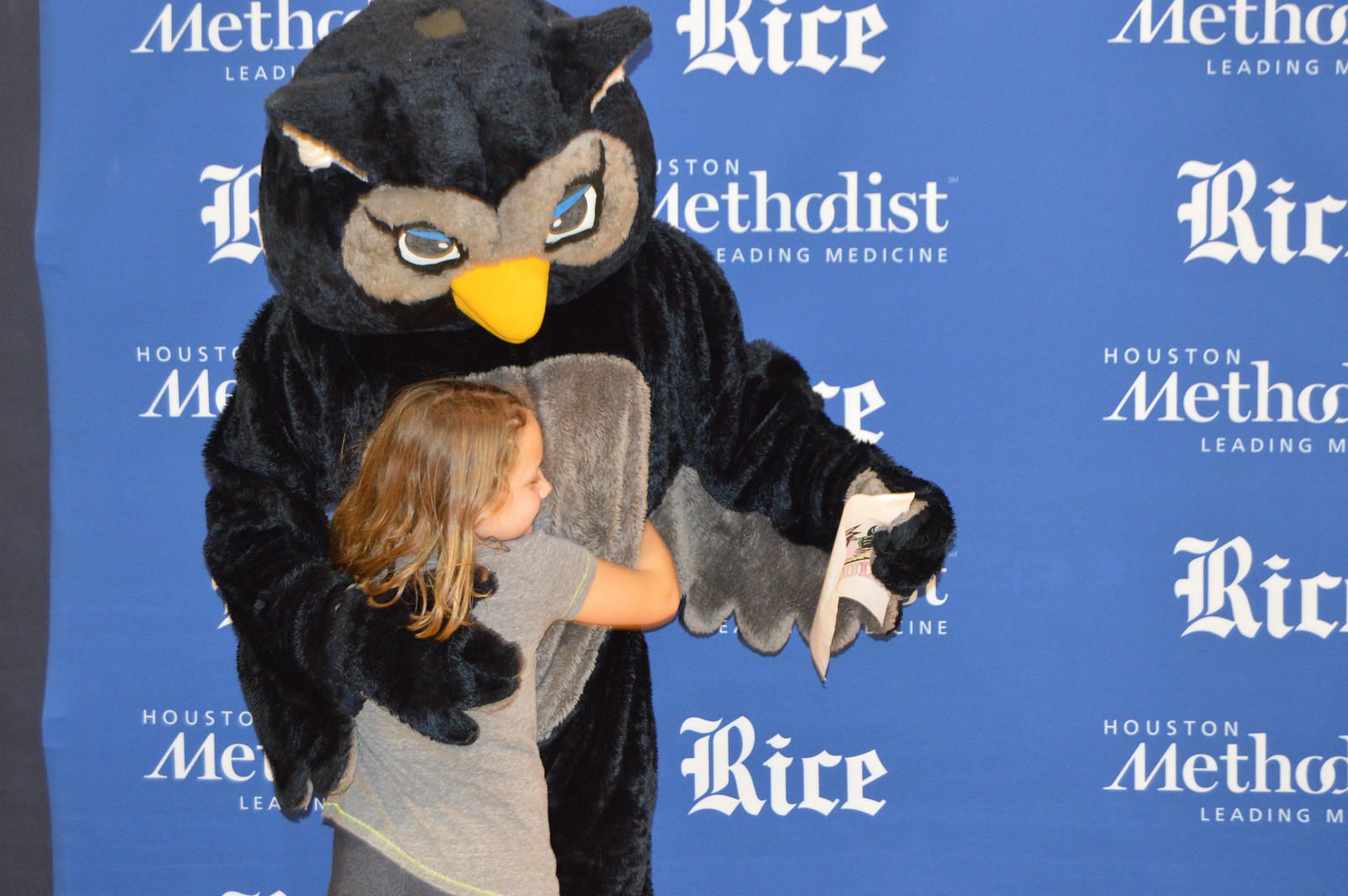This detailed color photograph, set indoors, features an adult dressed in a large, elaborate owl mascot costume. The owl has a white body with a gray belly, black ears with white inner ear, black eyes with blue eyelids, and a beak that appears to be a mix of yellow and orange hues. The mascot is holding a white booklet in its left hand while tenderly embracing a young girl, approximately seven or eight years old, with its right arm. The young girl, who has medium-length brown hair, is wearing a gray t-shirt and darker gray sweatpants, and her face is gently pressed against the owl's gray belly. Behind them, a blue backdrop prominently displays the words "Rice" and "Houston Methodist Leading Medicine," suggesting affiliations with these institutions, either hospitals or universities.